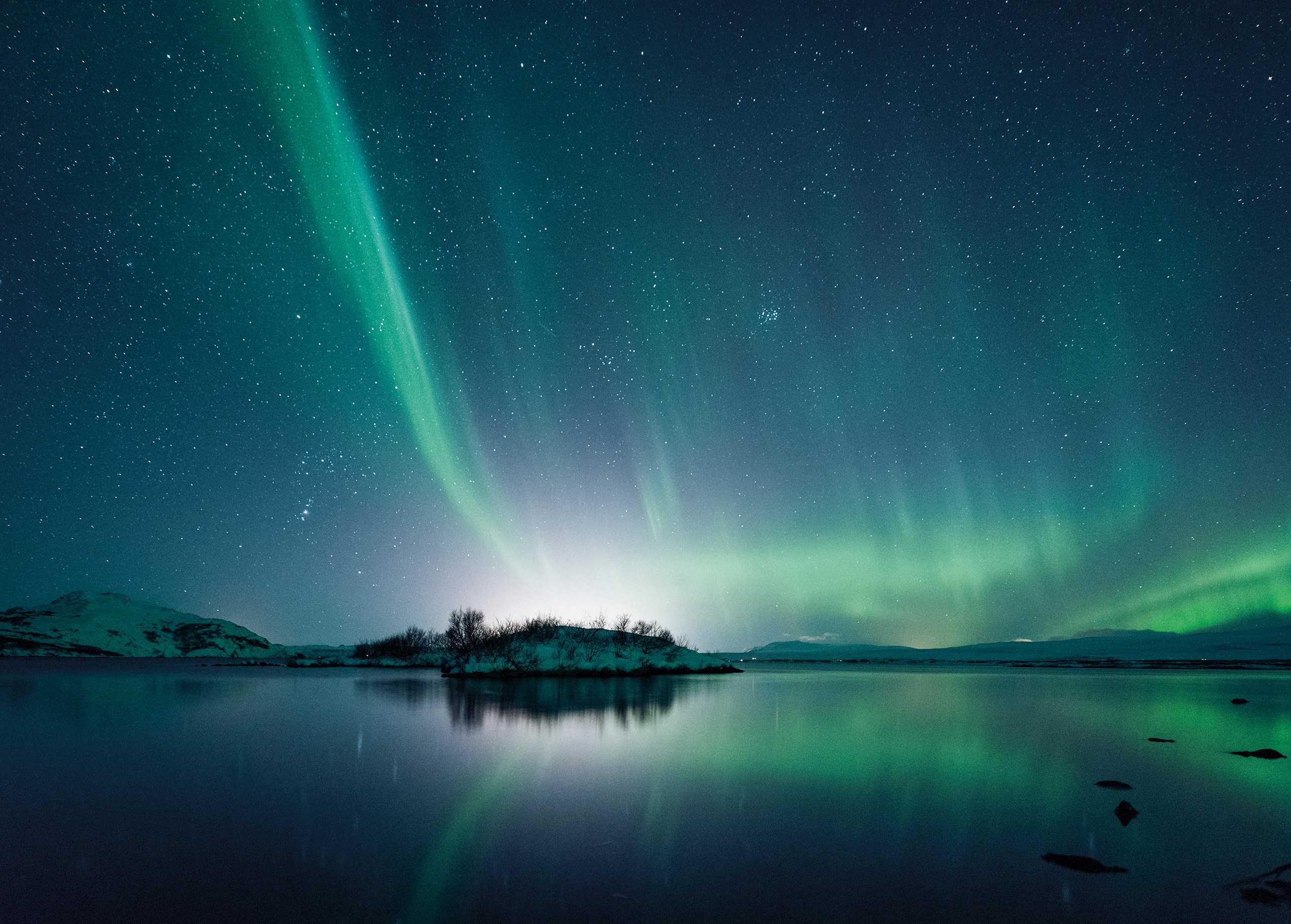This breathtaking image captures a serene, glassy lake with a few rocks scattered along its right side. A small island adorned with petite trees sits in the mid-range of the scene. In the distance, rolling, snow-covered hills create a picturesque backdrop. The night sky is densely filled with innumerable stars, their abundance making it difficult to discern specific constellations. Dominating the heavens, the northern lights dance vibrantly, their shimmering green hues reflected perfectly in the lake's smooth surface. The absence of light pollution enhances the clarity and brilliance of the aurora, making this a truly mesmerizing natural spectacle.